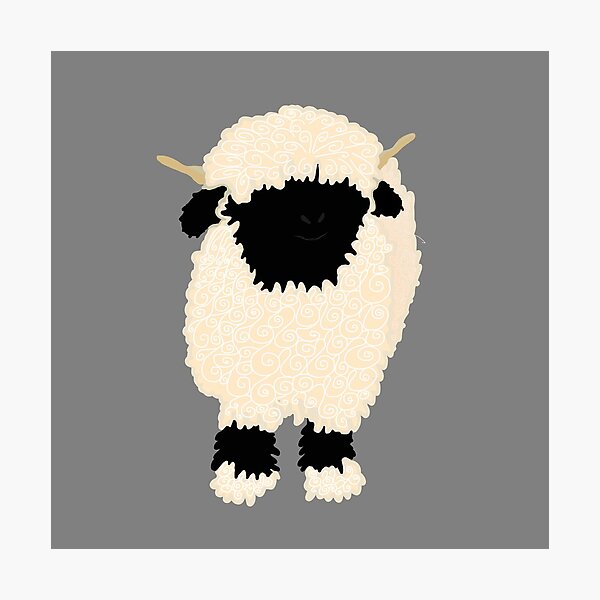The image is a piece of art depicting a sheep, designed with a mixed-media style that resembles a paper cutout collage. It is framed by a light grey border that is visible on every edge. The inner section features a solid dark grey, rectangular background. The sheep is centered and facing forward. Its body, rendered in a tan-colored oval shape, is adorned with white, swirled lines indicating thick, curly wool. The sheep has distinct black ears on either side of its head, and thin, upward-pointing white horns. Its legs are black, transitioning into white feet. Notably, its face is also black, presented as a featureless blob. This simple yet striking depiction combines the visual appeal of minimalist drawing with the dimensionality of a paper cutout art piece.